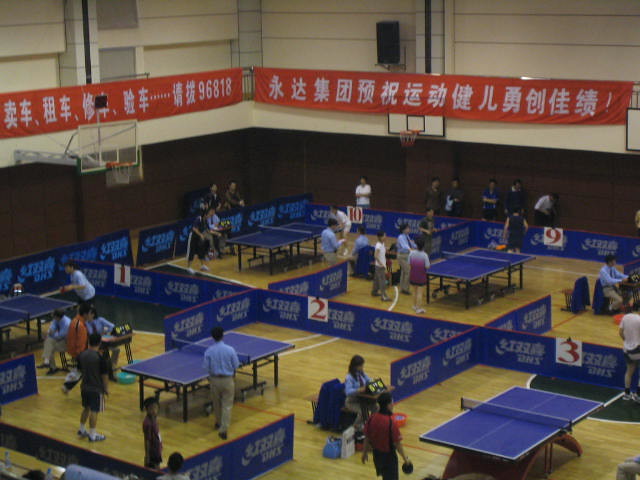The photograph, taken from an aerial perspective, captures a lively table tennis competition set inside a gymnasium. The gym floor is meticulously arranged with five distinct playing areas, each marked by short blue partitions adorned with text and numbered for clarity. In each section, there's a judge seated at a small desk, identifiable by their white shirts and tan pants. The competitors, both girls and guys, are actively engaged in games while a modest number of spectators line the sides, observing the matches.

The gym's walls feature a dual color scheme, brown on the bottom half and cream above, punctuated by multiple basketball hoops. A prominent red banner with Asian characters, likely Mandarin, and some numbers runs along the upper part of the wall, adding an international flair to the setting. The blue ping-pong tables, which appear to be folding types, are the focal points of the image. The scene has the characteristic buzz of a well-organized sporting event, with around 15 to 20 people either playing, judging, or milling about the gymnasium.